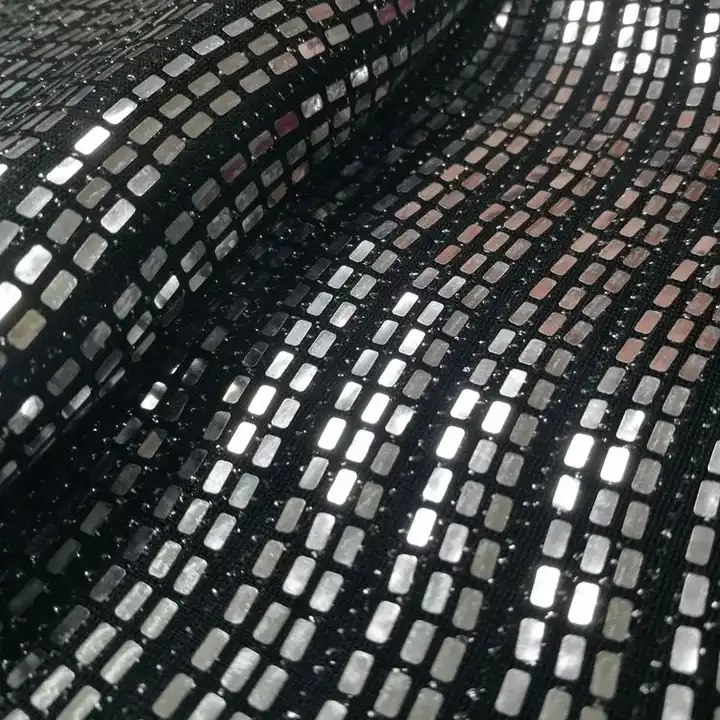The image showcases a detailed, mid-range view of an intriguing black knit or woven fabric. This fabric features symmetrical rows of shiny, mirrored rectangular spangles with rounded corners, which are meticulously sewn onto the surface. The spangles, resembling tiny roads, are uniformly aligned in groups of three, separated by small gaps, creating a rhythmic pattern across the fabric. In the upper left-hand corner of the image, the fabric is folded over itself, introducing a visible fold line and a rounded section where the top of the fabric overlaps the bottom. The black thread used to attach the spangles accentuates the shiny, reflective quality of the embedded metallic pieces, contributing to the overall dimensional and textured appearance of the fabric. There's an observed stretch component, hinting at the fabric's flexibility and dynamic texture.